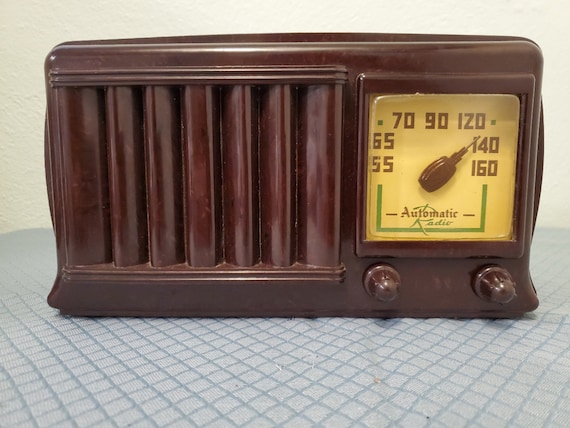This is a detailed color photograph of an antique clock radio, noted for its polished brown bakelite casing which gleams under the light. The radio, about the size of a large toaster, rests on a light blue cloth with a checkered pattern, the pale grey background adding a subtle contrast. The design features slats on the left side that lend it a radiator-like appearance, while on the right side, there are two control knobs and an adjacent display.

The display is distinguished by a spiral arrangement of numbers in a light yellow hue, ranging from 55 to 160, with a needle currently pointing at 140. The dial has significant and colorful markings, including two green dots and a green line that extends around the perimeter of the dial. Above the numbers, the words "Chromatic Radio" are printed, with "Automatic Radio" at the lower right, where 'Automatic' matches the radio's brown color and 'Radio' is in green, echoing the detailing on the dial. This image captures the essence of vintage design and craftsmanship, portraying an era where functionality met intricate aesthetic detail.